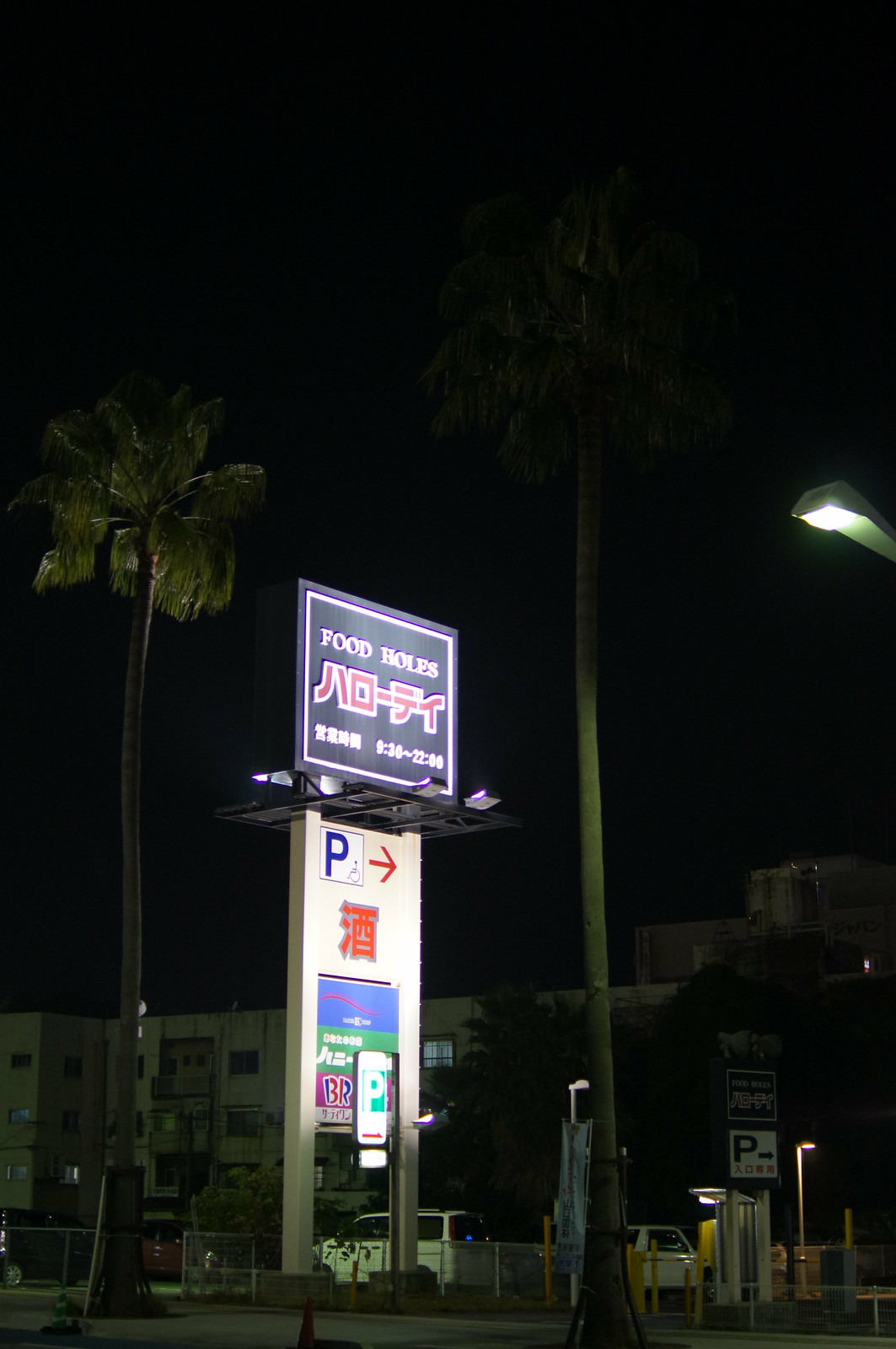This nighttime photograph captures a small, billboard-like sign illuminated by streetlights. The scene features a prominent parking direction sign, marked with a white rectangle containing a red arrow pointing to the right and the letter "P," alongside symbols and logos, including that of Baskin-Robbins. Above this is a lit black panel with white trim displaying the text "Food Hours" in English, alongside what might be Korean or Japanese characters, and hours listed as "9:30 to 22:00." The background shows the silhouettes of tall palm trees, residential buildings, and a couple of white cars parked near a roadway. The upper part of the image fades into darkness, adding to the night-time ambiance.